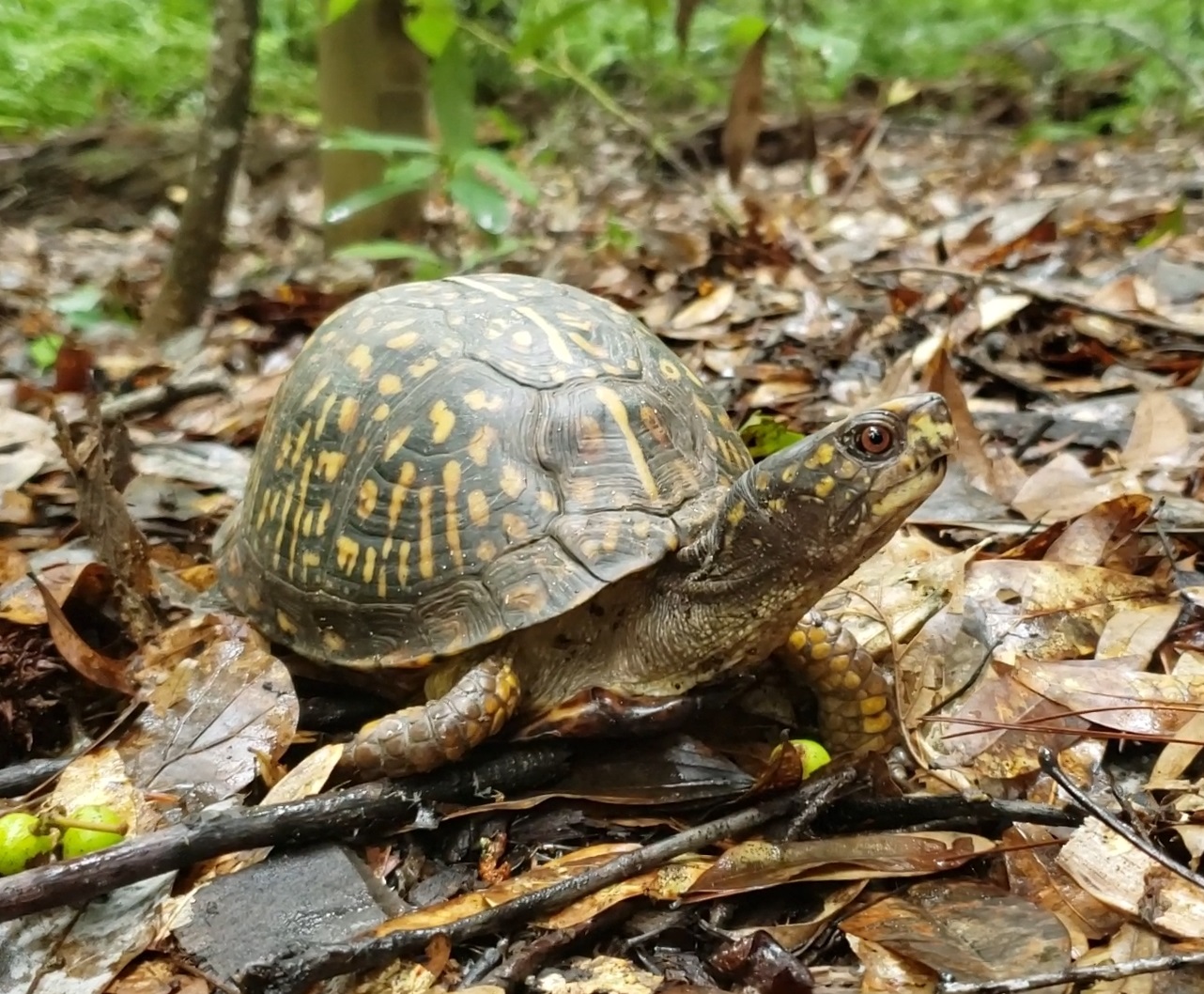In the image, a medium-sized turtle is captured in a forest setting, surrounded by a dense layer of dead leaves and sticks on the ground. The turtle, bearing a dome-like, greenish-gray shell with yellow spots and vertical stripes, somewhat reminiscent of an old German helmet, is positioned prominently in the foreground. Its head, adorned with light green skin and yellow spots, is extended and turned slightly upward and to the right, revealing its light brown, almost hazel, eyes in a semi-profile view. The turtle's front legs, which have a wrinkly, scaly appearance, are clearly visible as it seems to be walking towards its gaze. Scattered among the leaves are small bright green berries, possibly the turtle's intended target. The background features stereotypical forest elements, including some slightly out-of-focus green bushes and trees.